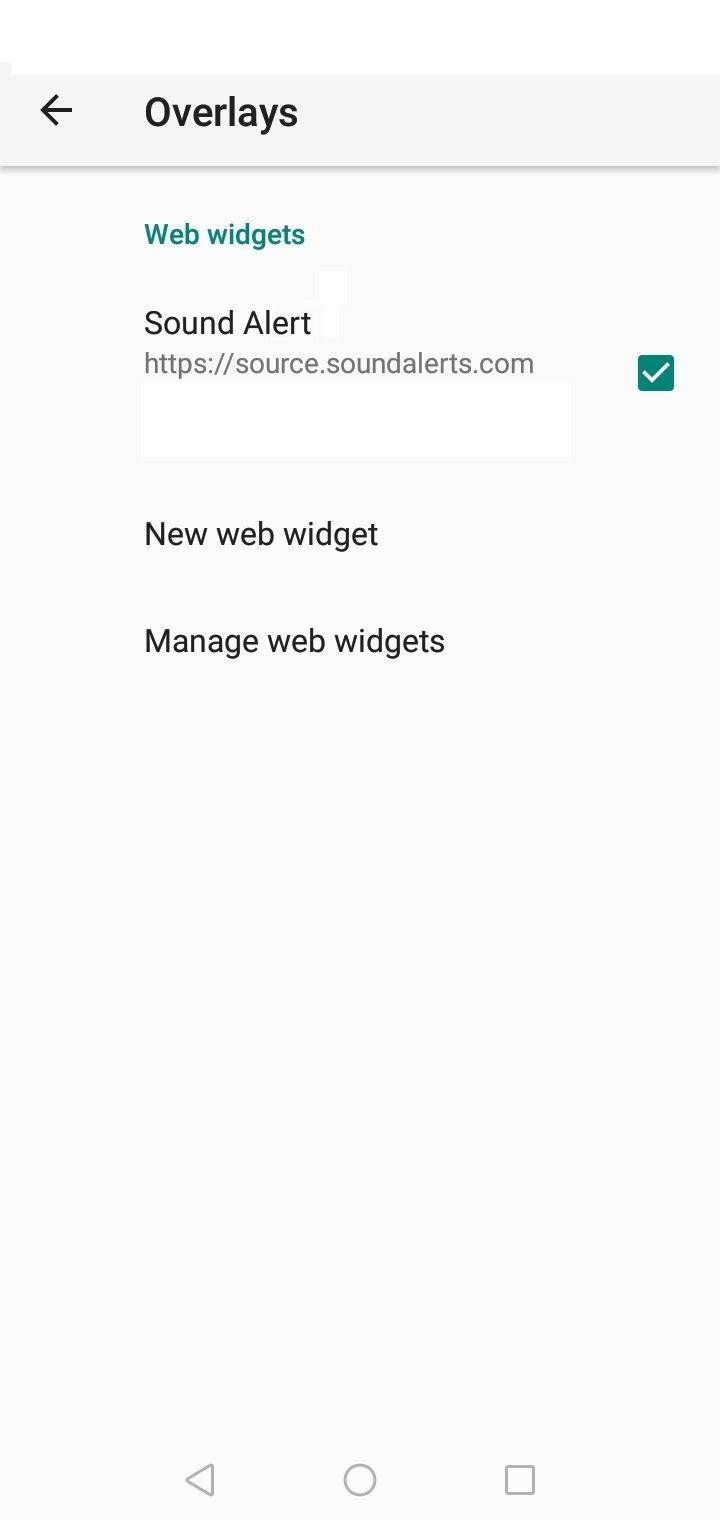A screenshot is displayed on a cell phone screen with a simple, white background. At the top, there's a light gray shaded bar featuring a black arrow pointing to the left and bold text reading "Overlays." Beneath this bar, there's a faint line. Below the line, the phrase "Web Widgets" is written in blue. Under "Web Widgets," the text "Sound Alert" is listed, accompanied by a URL: "HTTPS source.soundalerts.com." To the right of this URL, there's a blue square containing a white checkmark. Further down, the words "New Web Widget" appear in black text, followed by "Manage Web Widgets," also in black. At the bottom of the screen, a similar black arrow points to the left, alongside a circular button in the center and a hollow square icon in the bottom right corner.